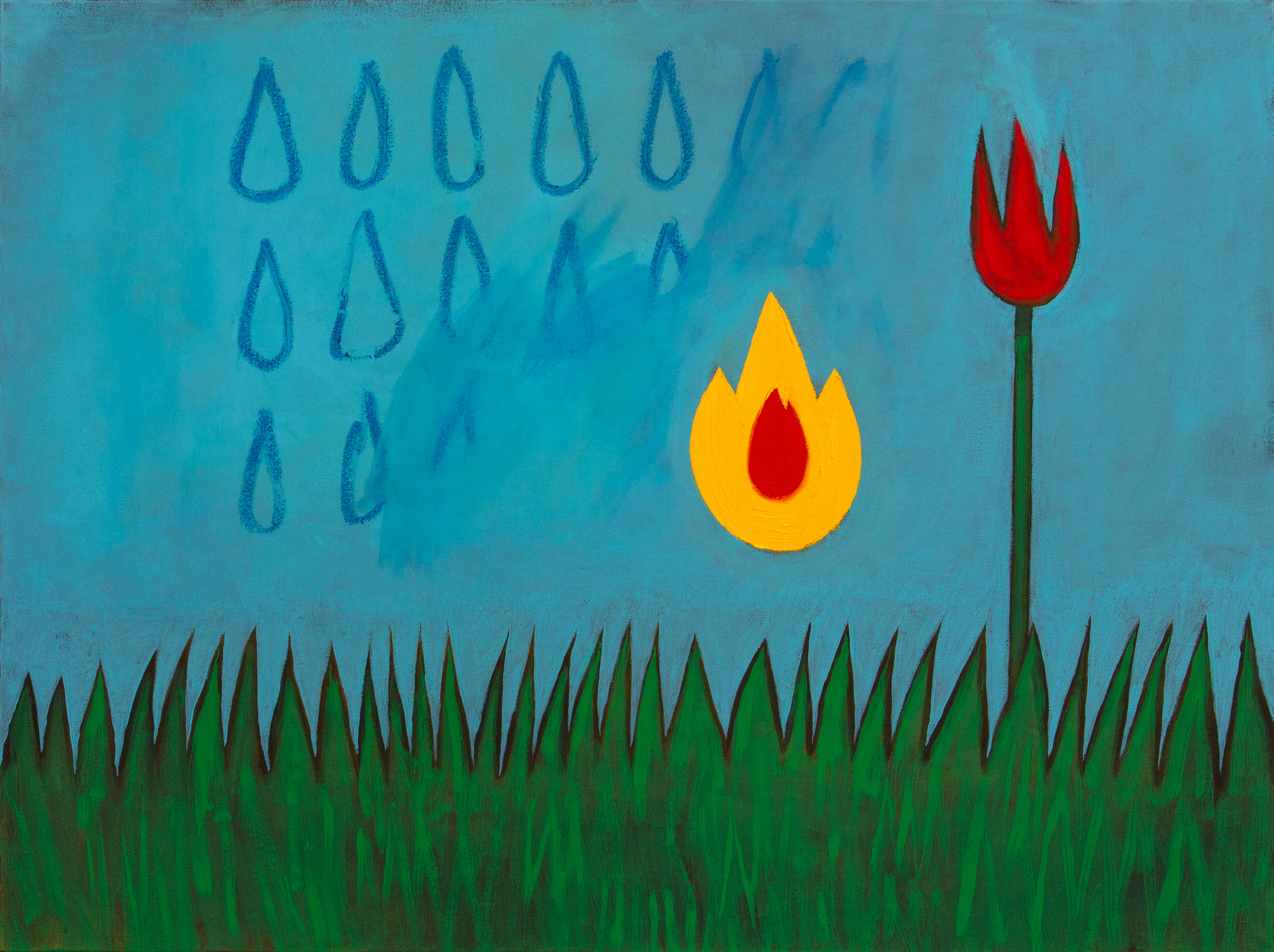This image is an abstract-style painting, characterized by its childlike simplicity yet intricately detailed elements. The scene features a vivid depiction of thick, sharp blades of green grass at the bottom, with each blade forming pointed tips and surrounded by a black border. Rising from amidst the grass on the right-hand side is a singular green stem supporting a vibrant red tulip.

To the left of the tulip, a striking teardrop-shaped flame with a yellow exterior and an elongated red core floats in the middle of a swirling blue sky, unattached and ethereal. The background sky consists of varying shades of blue, intricately blended to create a swirling effect.

Interspersed within this blue expanse are numerous large raindrops arranged in three staggered rows. The raindrops are meticulously ordered: the top row has five complete raindrops with two partially covered by the blue paint, the second row comprises four complete raindrops with one partly erased, and the bottom row has two fully depicted raindrops and one partially obscured. The raindrops, initially distinct on the left, gradually fade into the swirling blue background as they extend towards the right, creating a sense of dynamic motion and interaction between the elements.